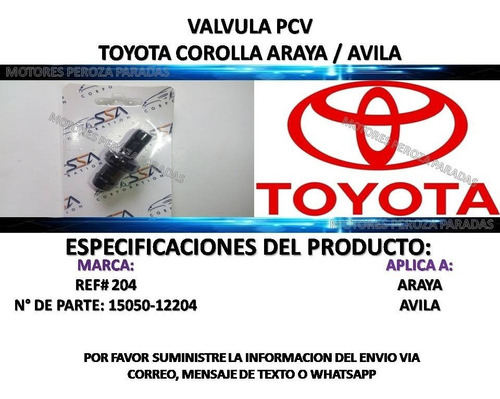The image features a packaged auto part for a Toyota Corolla, possibly a spark plug, prominently displayed in the left half of the frame. The part, black in color, is enclosed in a plastic container emblazoned with the SSA logo. The packaging includes text in Spanish, indicating it is a 'Valvula PCV' suitable for 'Toyota Corolla Araya/Avila'. 

On the right side of the image, the red Toyota logo along with the word 'Toyota' is prominently displayed. Below this, the text 'Especificaciones del Producto' is visible, followed by 'Marca' in purple, and 'Aplica A' indicating the part's applicability to specific car models. The reference number '204' and part number '15050-1204 Araya Avila' are listed below. At the bottom, there is a request in Spanish: 'Por favor, suministre la información del envío via correo, mensaje de texto o WhatsApp' (Please provide the shipping information via email, text message, or WhatsApp).